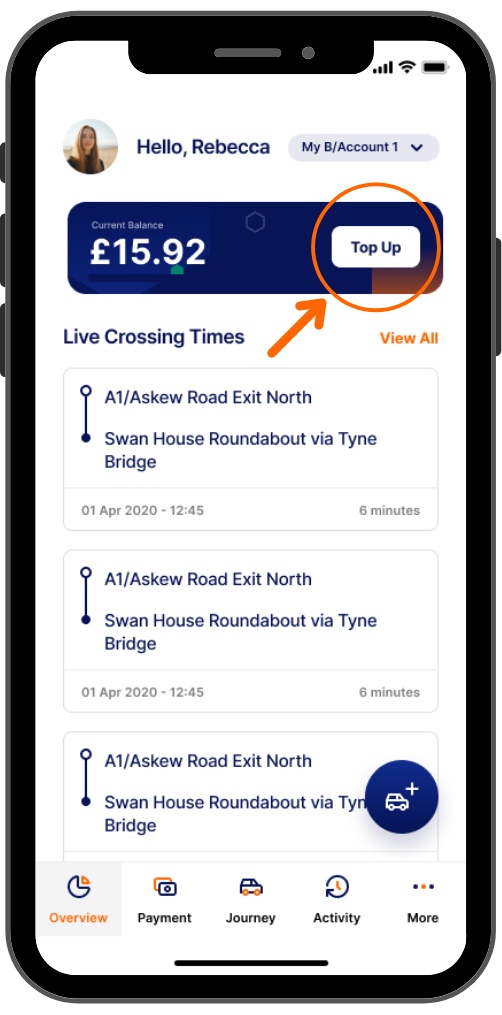The image depicts a cell phone screen with a black border. In the top right corner, a set of icons indicates strong cellular reception with four bars, a connected Wi-Fi signal, and a nearly full battery. 

On the left side of the screen, there is a circular profile picture of a young Caucasian woman with long brown hair. Next to the image, text reads, "Hello Rebecca. My B/Account One." 

Below this section, in a rectangular box, it states "Current balance: £15.92" with an adjacent "Top Up" button highlighted with an orange circle and a pointing arrow.

Further down, under the heading "Live Crossing Times - View All," detailed information about several routes is laid out as follows:
- "A1/Askew Road Exit North, Swan House Roundabout via Tyne Bridge, 01 April 2020, 12:45, 6 minutes."
- This route information is repeated twice more with identical details.

A blue circle containing a vehicle icon and a plus sign is also present within this section.

At the bottom of the screen, five navigation icons are displayed:
1. A Pac-Man-like icon with an open mouth labeled "Overview."
2. Two stacked rectangles, labeled "Payment."
3. An icon of a vehicle, labeled "Journey."
4. A circular arrow icon, where the arrow constitutes both the border and the edge, labeled "Activity."
5. Three dots in dark blue, yellow-orange, and another dark blue, labeled "More."

This detailed description effectively captures the various elements present on the cell phone screen.